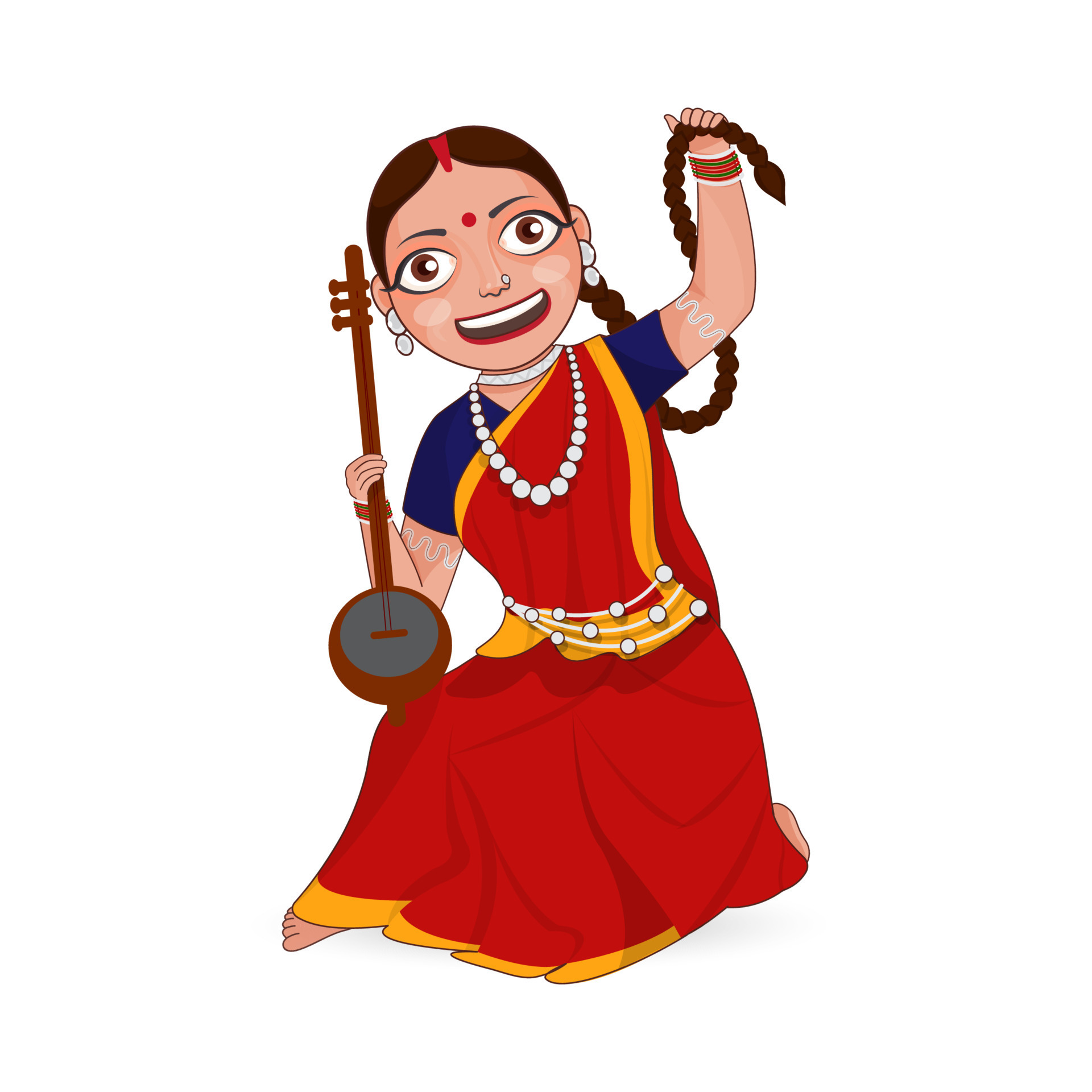The image depicts a vibrant, hand-drawn cartoon of a young Hindu woman, evident by the red dot (Bindi) on her forehead, often associated with Hinduism and South Asian culture. She has a cheerful expression, with brown eyes and long brown hair intricately braided, which she holds up with her left hand adorned with colorful red and green bangles. Her attire features a rich red sari with golden stripes along the hem and sides, under which she wears a dark blue blouse. She is barefoot and kneeling on one knee. She wears a variety of jewelry, including larger earrings, a pearl necklace, a choker, and a nose piercing. In her right hand, she holds a small, brown stringed instrument resembling a banjo with a blue-green center and a simple, long neck. The detailed artwork captures the cultural essence and joyful spirit of the character, blending traditional elements with artistic flair.